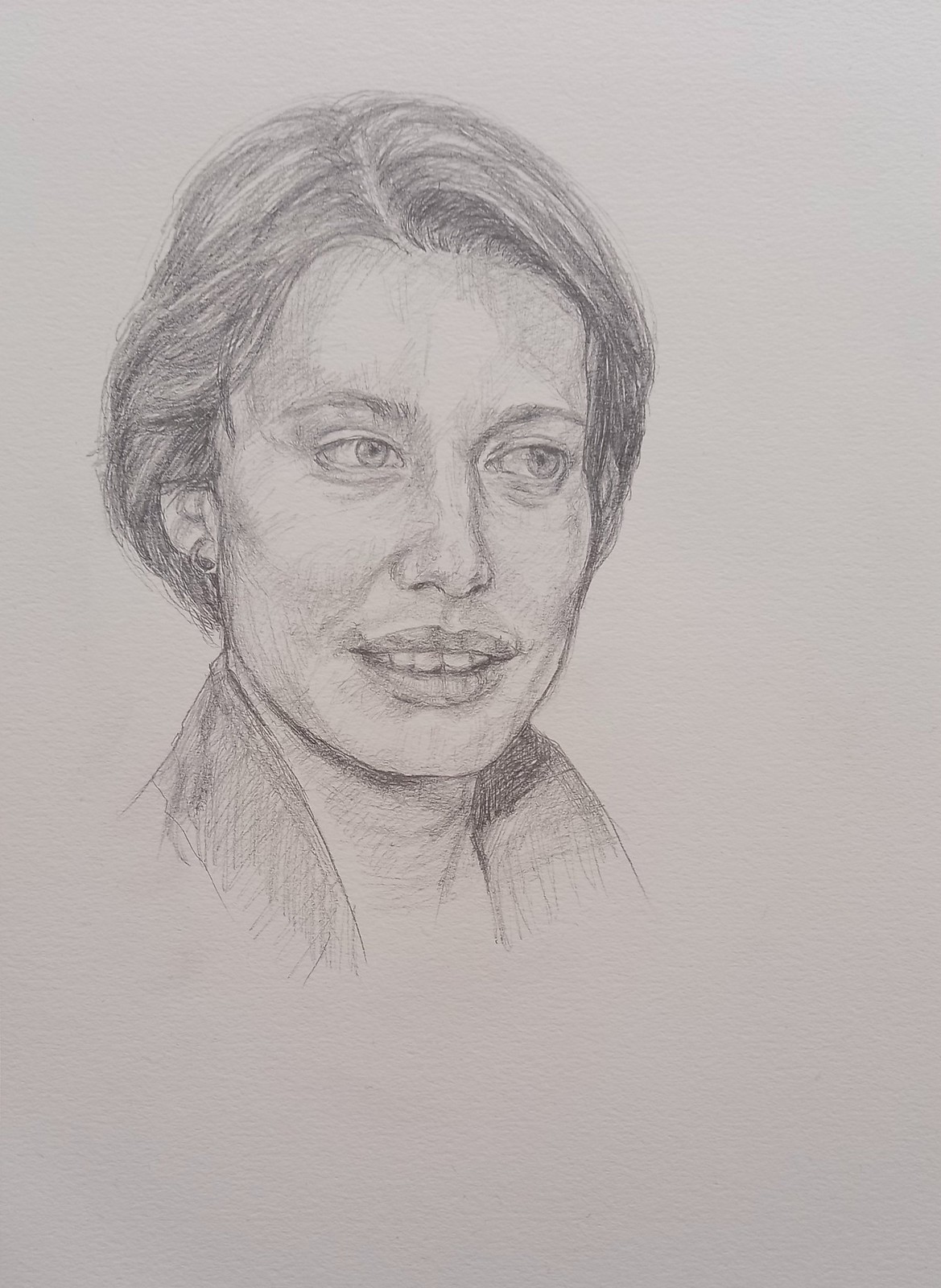This detailed pencil sketch appears to be a self-portrait of a woman, set against a very light gray background. The artist has depicted herself with a subtle elegance that hints at a certain maturity, possibly in her 30s or a bit older. Her hair, which might be gray, is parted to the side and falls just below her ears. The woman's expression is reminiscent of the iconic Mona Lisa, with a gentle, almost enigmatic half-smile that reveals a hint of her teeth. Her gaze is directed at an angle, looking away from the viewer, which adds a sense of introspection to the portrait. She is adorned with simple earrings and is dressed in a garment with a prominent collar that rises halfway up her neck, adding a touch of sophistication to the overall composition.